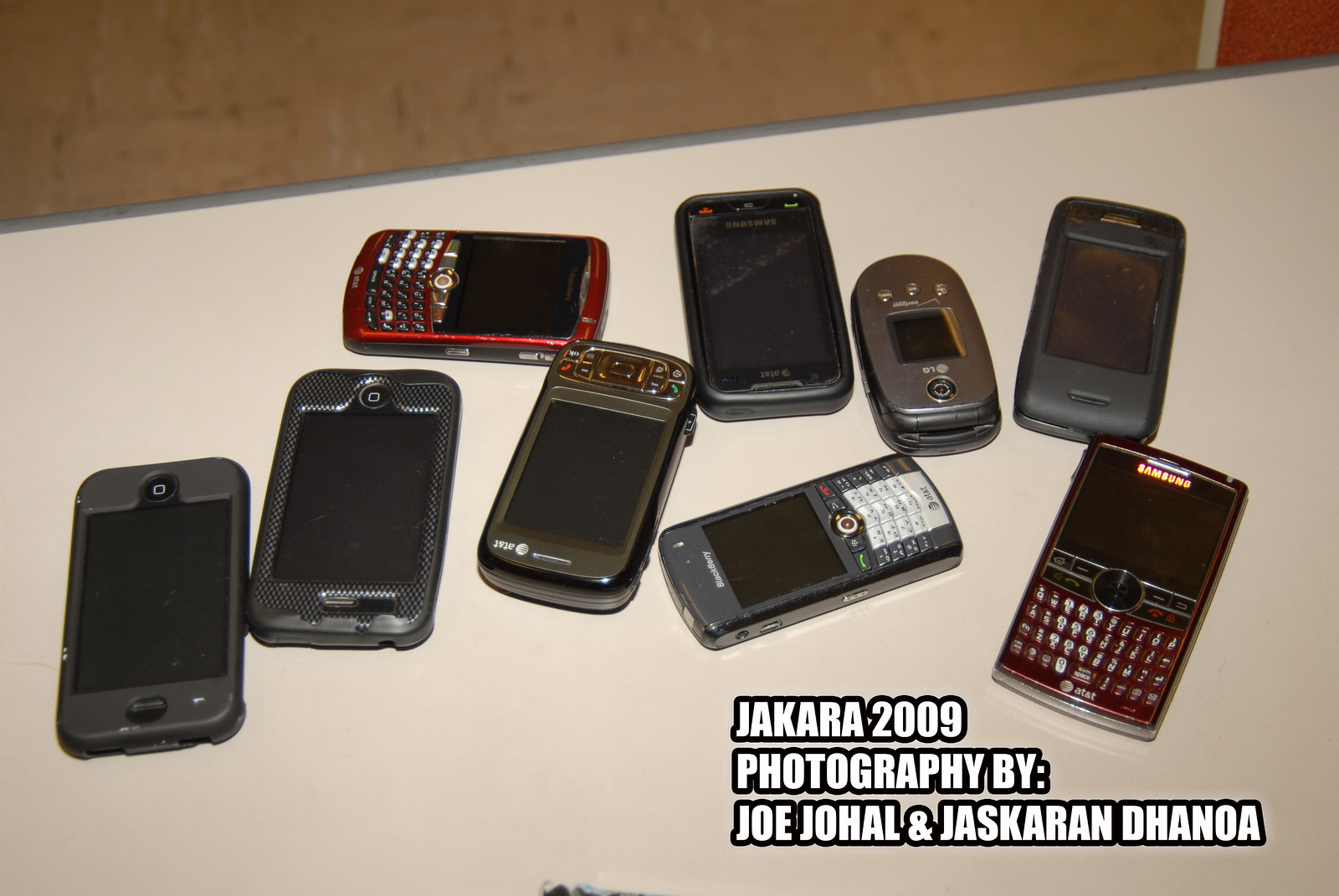The image features a diverse collection of cell phones predominantly from the late 90s to early 2010s, displayed on a beige table. The assortment includes mainly Samsung, BlackBerry, and LG models. Notably, there's a burgundy Samsung phone resembling a BlackBerry with "ATT" inscribed on it, an actual red BlackBerry, a black BlackBerry, and various flip phones including an LG model. Also present are two small, brick-like phones and two others with home buttons. Among the smartphones, three have chunky black covers and visible keyboards, while some are characterized by their vibrant red or maroon colors, contrasting the predominantly black array. In the backdrop, a brown wall can be seen. The image is captioned at the bottom with "Jakara 2009, Photography by Joe Jahal and Jaskeran Danoa."